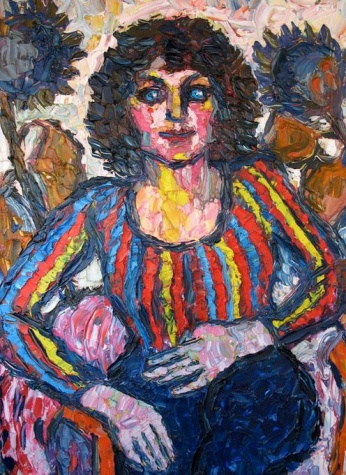This vivid and modern-style painting depicts a young woman positioned centrally, taking up most of the image. Her strikingly blue eyes, devoid of any white, are a dominant feature, alongside her short, possibly curly brown hair with hints of blue. She sports a scoop-neck shirt with bold, vivid blue, red, and yellow stripes on the bodice and long sleeves. Her fair skin is painted with a mix of colors, including yellow, red, and touches of white, giving it a unique, multi-tonal appearance. 

The woman’s lips are painted a bright red, contrasting her rosy cheeks. One of her hands rests on her hip while the other covers her stomach. She appears to be wearing blue pants. The background is minimal but features two large blue flowers or sunflowers on either side of her. Additional elements, possibly mountains or decorative designs in yellow, contribute to the intricate backdrop. This detailed and colorful painting would be a fitting piece for an art show or museum exhibition, bringing to life its central figure with a joyful expression.